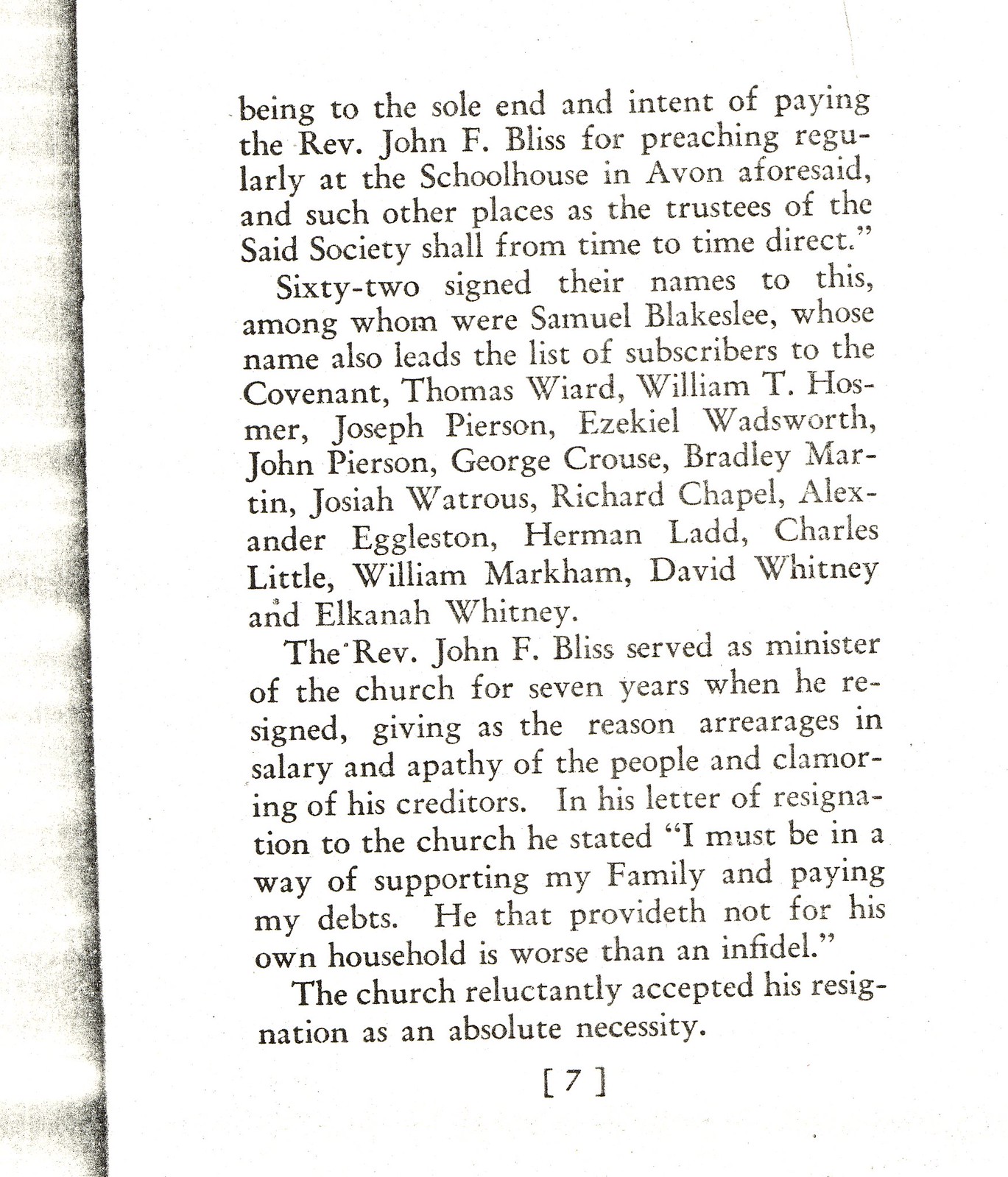This image displays a scanned page, marked as page seven, from an old book. The visible text details an account concerning the Reverend John F. Bliss. The passage begins by acknowledging the intent to compensate Reverend Bliss for his regular preaching at the schoolhouse in Avon and other locations as directed by the trustees. A total of 62 individuals signed their names in agreement to this intent, including notable names such as Samuel Blakeslee, Thomas Wyatt, William T. Hosmer, Joseph Pearson, Ezekiel Wadsworth, John Pearson, George Kraus, Bradley Martin, Josiah Watrous, Richard Chappell, Alexander Eggleston, Herman Ladd, Charles Little, William Markham, David Whitney, and Elkana Whitney. Despite his services, Reverend Bliss resigned after seven years due to unpaid salary, community apathy, and pressure from creditors. In his resignation letter, he emphasized the necessity of supporting his family and paying his debts by quoting, "He that provideth not for his own household is worse than an infidel." The church reluctantly accepted his resignation. The scan also faintly shows part of the adjacent page on the left.